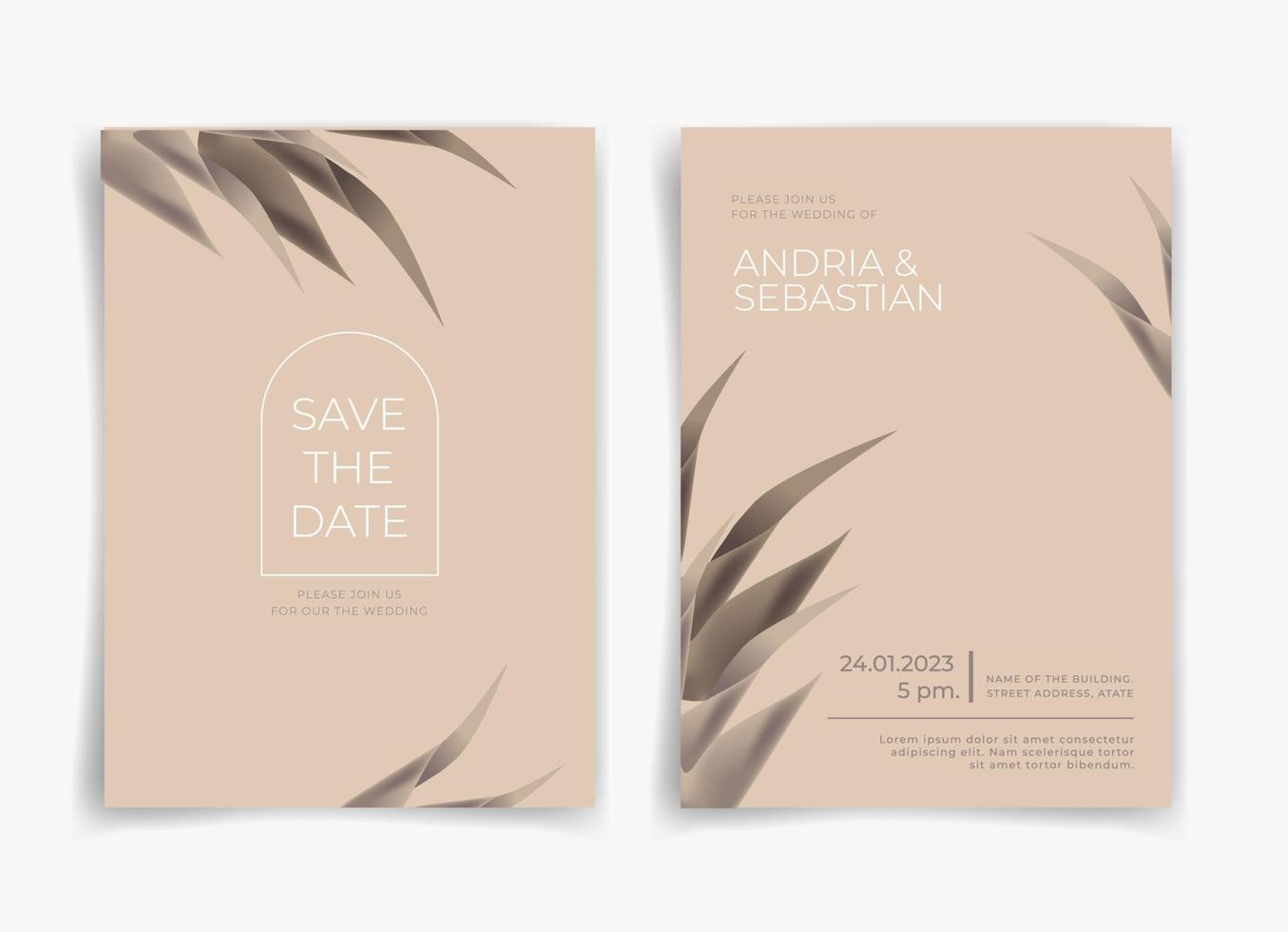The image displays a mockup of a wedding invitation card, showcasing both the front and back of the design. The card features a soft pink or beige background with delicate gray plant fronds adorning the top and bottom edges. On the left side, which likely represents the front of the invitation, there is an arched window outlined in white, containing the text "SAVE THE DATE" in white. Below the window, dark text reads "please join us for our the wedding," indicating a noticeable typo. The right side of the image, presumably the back or inside of the card, continues with the same background and design elements. The upper left contains the phrase "please join us for the wedding of" in dark text, followed by the names "Adria & Sebastian" in larger white font. The bottom right corner details the event information in black lettering: "24.01.2023, 5 PM," followed by a large black strike-through line and placeholder text in Latin, indicating where the venue and address details would be.